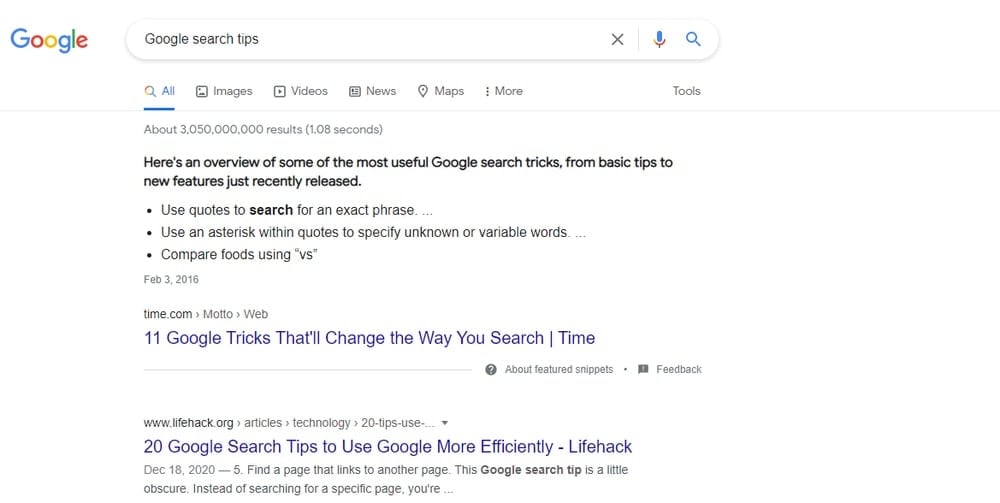The image displays a screenshot of a Google search results page. In the upper left corner, the Google logo is prominently featured. To the right, there is a search bar containing the query "Google Search Tips." Adjacent to the search bar, on the right side, there are three icons: an X for closing, a microphone for voice search, and a magnifying glass for initiating the search.

Below the search bar, there is a navigation menu with various categories including "All," "Images," "Videos," "News," "Maps," and "More," with the "All" category underlined to indicate it is currently selected. The search results indicate approximately 3,050,000,000 results found in 1.08 seconds.

Beneath this, there is an introductory text stating, "Here is an overview of some of the most useful Google Search tricks from basic tips to new features just recently released." Following this text, three bullet points provide specific search tips:
1. Use quotes to search for an exact phrase.
2. Use an asterisk within quotes to specify unknown or variable words.
3. Compare foods using 'versus'.

Below the tips, two specific search results are highlighted:
1. A link to a TIME article titled "11 Google tricks that will change the way you search."
2. A link to a Lifehack article titled "20 Google Search Tips to Use Google More Efficiently" dated December 18, 2020. The description for this result begins with "Find a page that links to another page. This Google Search tip is a little obscure. Instead of searching for a specific page, your..." and then trails off with an ellipsis.